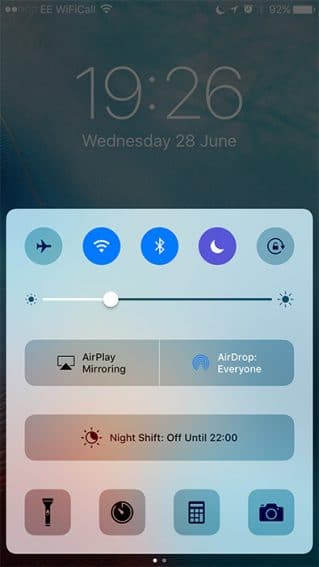The image displays a close-up view of a person's smartphone screen, meticulously showcasing various interface elements. The upper section of the screen has a bluish-grey background. In the top left corner, the phone indicates it is connected to the EE network and displays a Wi-Fi icon, suggesting an active wireless connection. On the right side, there is a crescent moon icon, possibly indicating Do Not Disturb mode, alongside several other icons and a battery indicator showing 92% charge remaining.

Centered beneath this, in a much larger font, the time is prominently displayed as 19:26, with the date below it, shown as Wednesday, June 28th. Just beneath the date, a light blue control panel is visible, featuring a series of icons. The top row includes an airplane symbol, a Wi-Fi signal icon, a Bluetooth symbol, what appears to be another moon icon, and a lock refresh icon. The screen brightness is set to approximately one-third of the available scale.

Further down, a panel dedicated to connectivity options is visible. On the left, labeled in black font, is the "AirPlay Mirroring" option. Opposite it, in white font, is the "AirDrop" option, marked as set to "Everyone." A separate panel below those indicates that "Night Shift" mode is off until 22:00.

Finally, at the bottom of the screen, there are four distinct icons. From left to right, they represent a flashlight, a stopwatch, a calculator, and a camera, each suggesting instant access to these utilities.

The overall image provides a comprehensive look at the various functionalities and settings available on the smartphone's user interface screen.